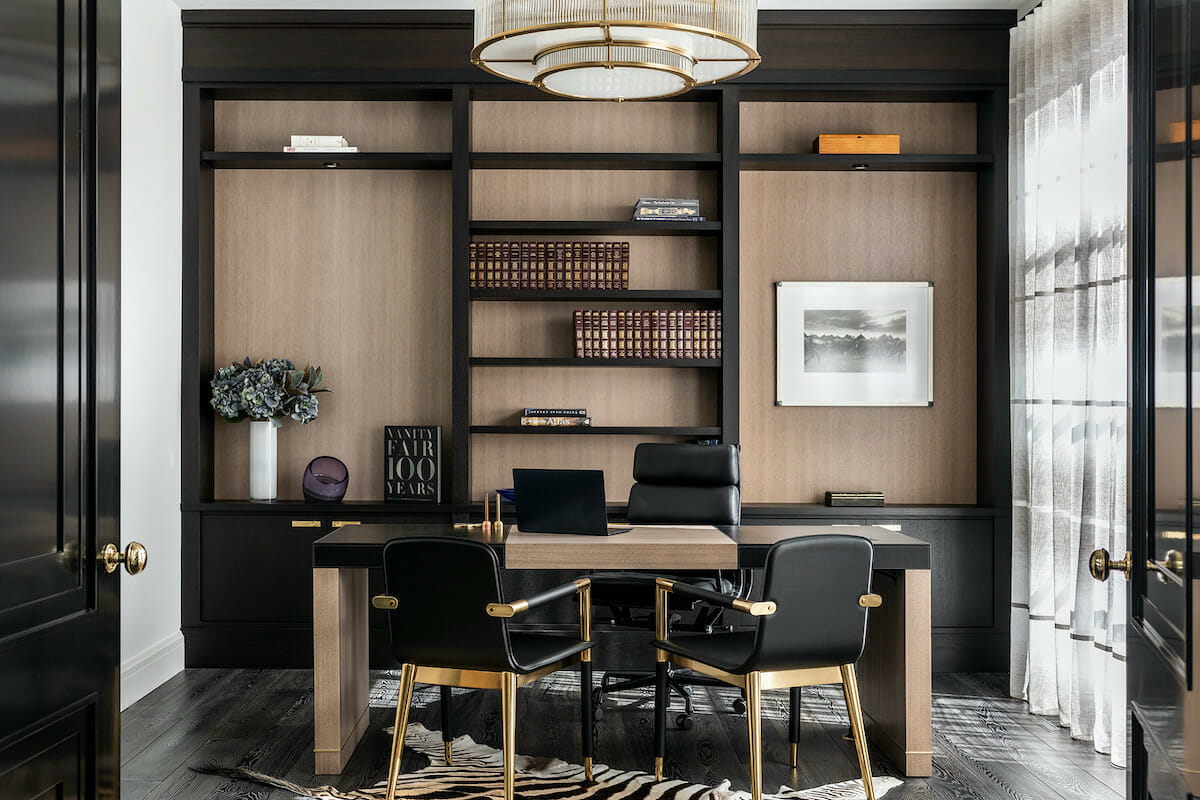This realistic, horizontally oriented photograph captures a meticulously designed modern office viewed through two open black doors with gold handles on either side, occupying the left and right 10% of the frame. The right side features a window draped with white curtains, letting in natural light. The left wall is painted white. Dominating the back wall is a built-in bookcase crafted from light brown wood with black cabinets and framework, holding approximately 20 to 30 books, a white vase with a plant, and a prominently displayed black book titled "Vanity Fair 100 Years" in gold font. A light brown desk with an open black laptop sits centrally, accompanied by a black manager's chair. In front of the desk are two black and gold chairs for visitors. The floor is covered in a distinctive zebra skin rug on top of rich black hardwood. A white portrait depicting mountains adds an artistic touch to the right side of the office.